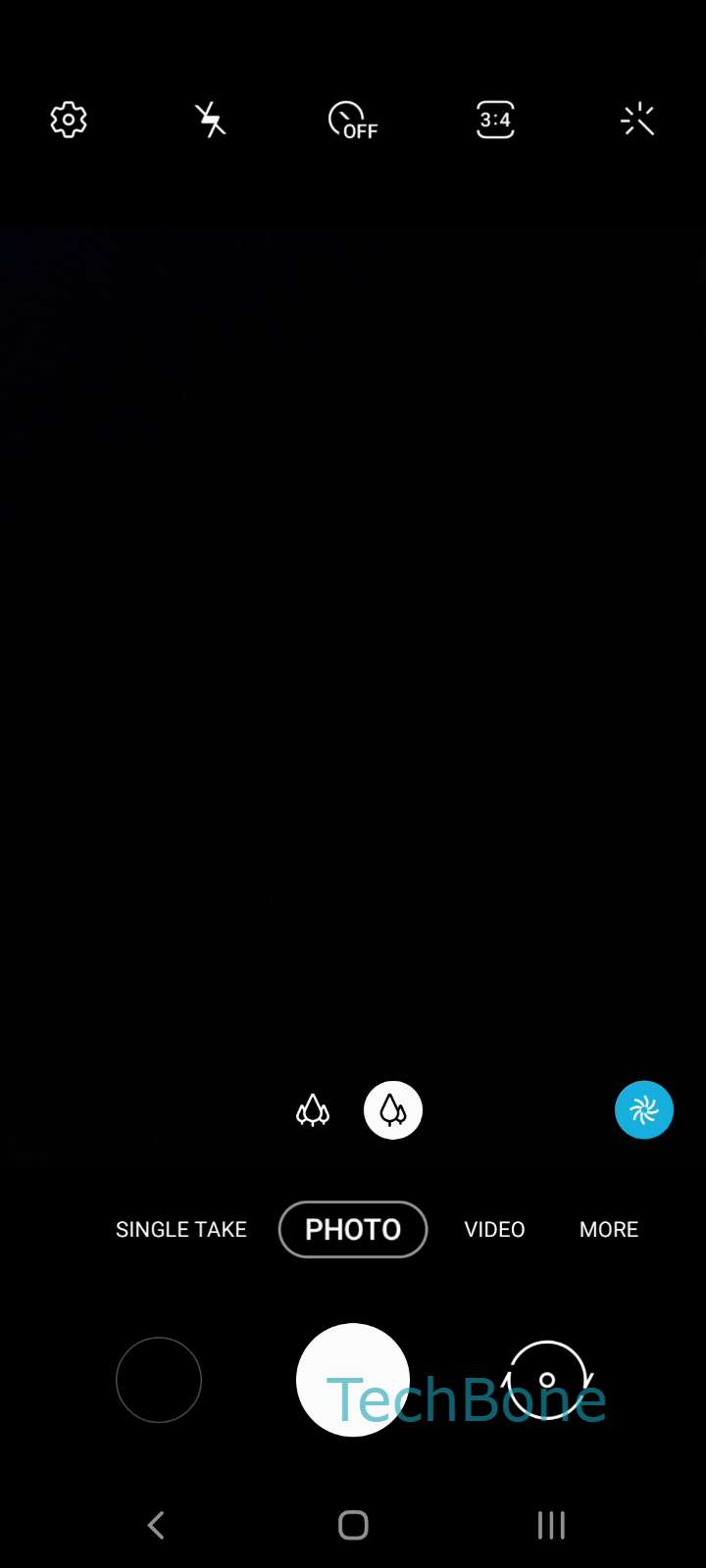The image appears to be a screenshot taken from someone's phone in camera mode. The background is completely jet black, devoid of any texture or dimension, giving a very flat, one-dimensional appearance. 

At the top of the screen, a series of white icons are visible, offering various camera settings. These include a flash icon with a line through it (indicating the flash is off), a timer labeled "off" with options for 3 and 4 seconds, and a brightness adjustment feature.

In the center of the screen, the jet-black background continues, with no discernible picture visible. At the bottom of the screen, several icons are displayed. These include an upside-down raindrop symbol and a prominent blue button featuring a white swirly design.

The bottom part of the screen allows for different capture modes, highlighted by the currently selected "Single Take" option. Other available modes include "Photo," "Video," and "More." Below these mode options are three circles. The first circle has a thin outline, the second is completely filled in white, and the third circle has a slightly thicker outline with an inner circle filled in with a tech-bone and seafoam green color.

Finally, at the very bottom, there is an arrow icon, a square, and three horizontal lines indicating additional options or menus.